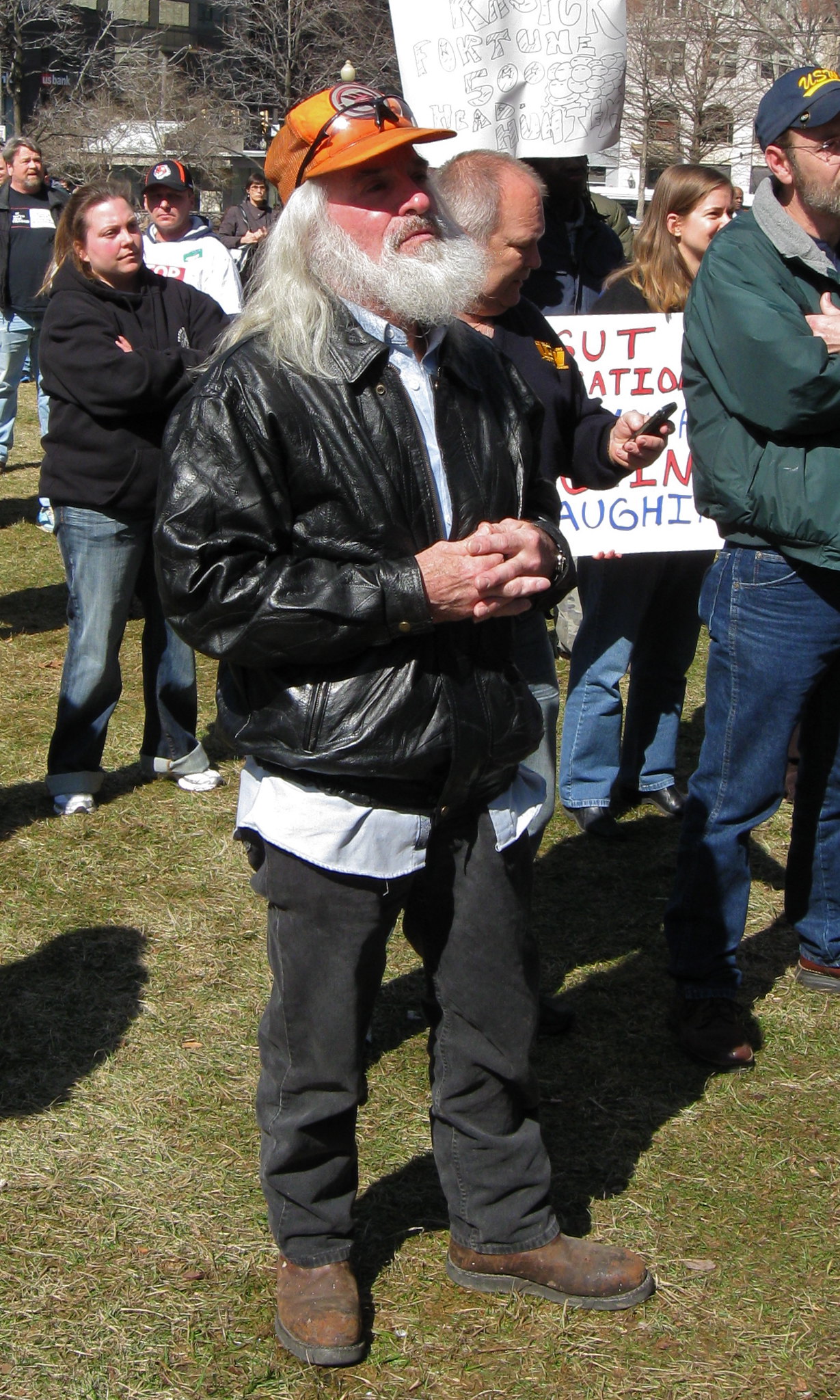The image depicts a peaceful protest in a park-like setting, with a diverse crowd holding various signs amidst trees and grass. Centered in the forefront stands a man, prominently wearing well-worn brown boots with black bottoms, black jeans, and a partially unzipped black leather jacket over a white button-up shirt. His distinctive orange baseball cap, adorned with black-rimmed safety glasses on its rim, sits above his long silver hair and gray beard. The crowd, dressed in an array of colors including black, brown, blue, green, yellow, white, and red, appears to be focused on something towards the right, possibly listening to a speaker. One notably held sign reads “Fortune 500 Head Hunt,” although many other signs are obscured by the people in front. The background features leafless trees and hints of nearby buildings, setting a scene of communal activism and solidarity.